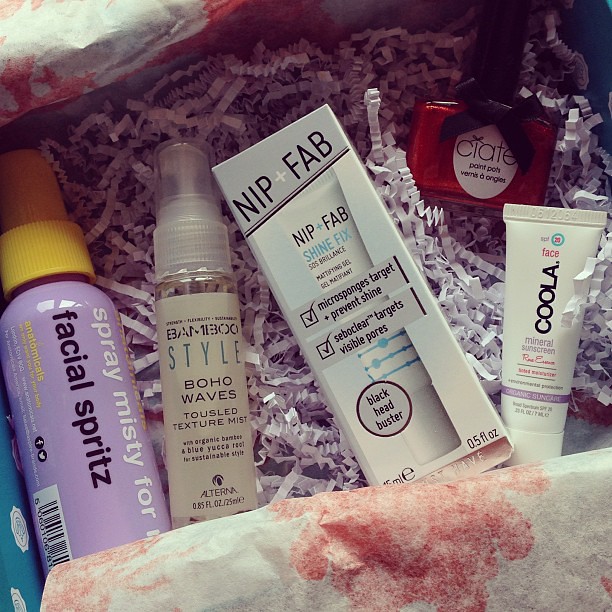"Captured in this image is an array of skincare products nestled in a gift box filled with decorative purple shredded paper and floral-patterned tissue paper. Starting from the left, there's a small, lavender-colored bottle with a yellow spray cap labeled 'Spray Misty for Facial Spritz.' Next to it is a sleek, brown bottle featuring a clear acrylic top and marked 'Bamboo Style Boho Waves Tousled Texture Mist.' Moving right, a white box prominently displays 'Nip + Fab Shine Fix,' which includes micro sponges that target and prevent shine, address visible pores, and tackle blackheads. Adjacent to this box is a tube of sunscreen held in a white container. Completing the collection is a vibrant red bottle of nail polish from the brand 'Ciaté,' adding a bold touch to the assortment of facial and skincare products. The entire ensemble is cushioned by the shredded paper for protection, creating a visually appealing and practical gift presentation."